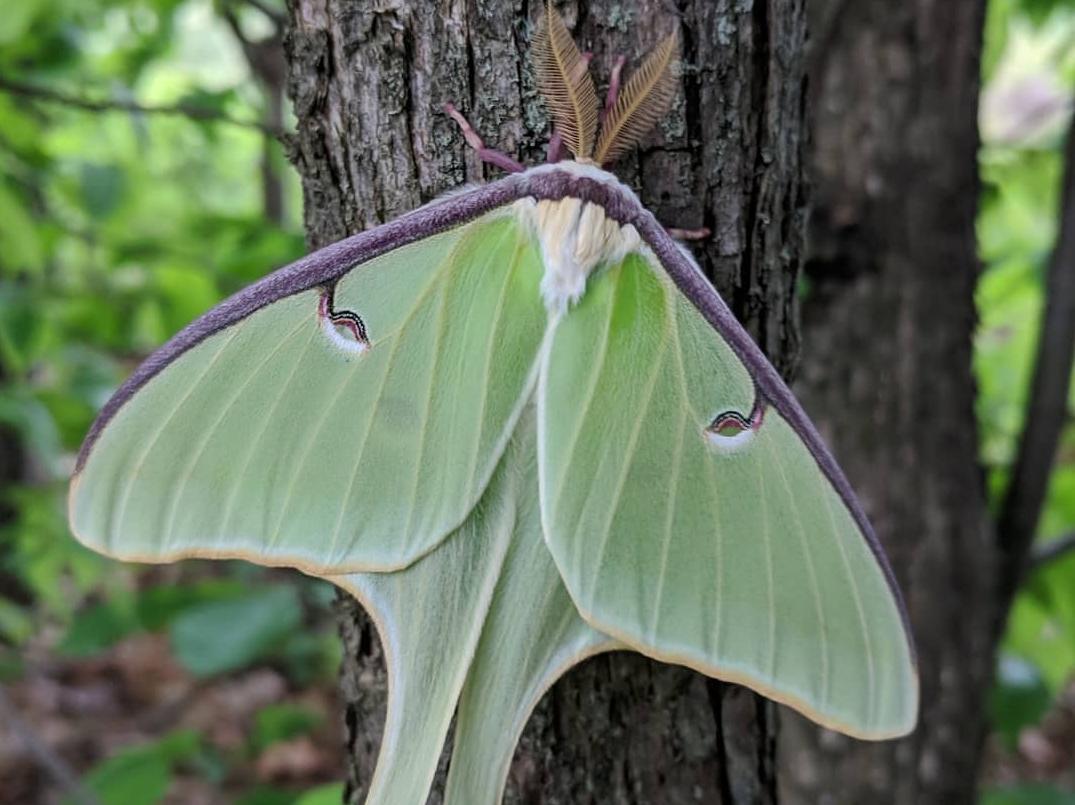This colour close-up photograph captures a strikingly detailed image of a large green Luna moth, prominently clinging to the dark bark of a small tree. The moth's semi-transparent wings, delicate and veined like leaves, display a light green hue with a purplish-brown fur-like border along the upper edge. Extending from the wings are long, kite-shaped tails, cropped just slightly at the bottom of the image. At the moth's head, two feathery, golden-brown fern-like antennae protrude, while a small patch of white fur lies just beneath them. The moth's slender legs grip the textured bark of the tree. The immediate foreground is sharply in focus, emphasizing the detailed textures of both the moth and tree bark. The out-of-focus background reveals a blurred forest and greenery, further accentuating the moth's grand presence in this natural setting.